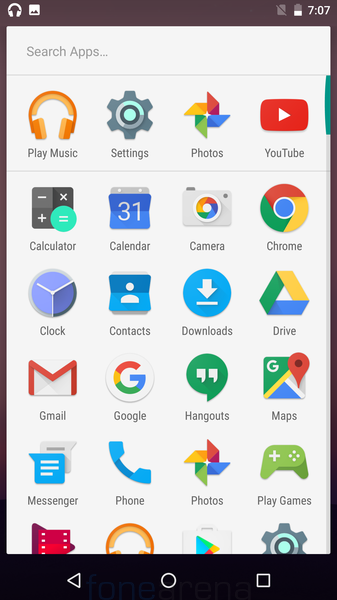This screenshot captures the home screen of an Android mobile phone, featuring a clean layout with a white background and a black border at the top. In the top-right corner, there are icons for headphones and photographs. The visible battery level is around 40%, and the time displayed is 7:07.

Dominating the screen are six rows and four columns of app icons, arranged neatly below a white search bar designed for quick app searches. Starting from the top left corner, the following apps are visible: Play Music, Settings, Photos, YouTube, Calculator, Calendar, Camera, Chrome, Clock, Contacts, Downloads, Drive, Gmail, Google, Hangouts, Maps, Messenger, Phone, Photos, Play Games, and Play Store. Unfortunately, two app icons are partially obscured, and their names cannot be fully discerned without scrolling.

The bottom of the screen features the classic Android navigation bar with a left-pointing triangle (Back button), a circle (Home button), and a square (Recent apps button), all set against a black border. The meticulous organization and familiar app icons make this a quintessential snapshot of an Android user’s home screen.